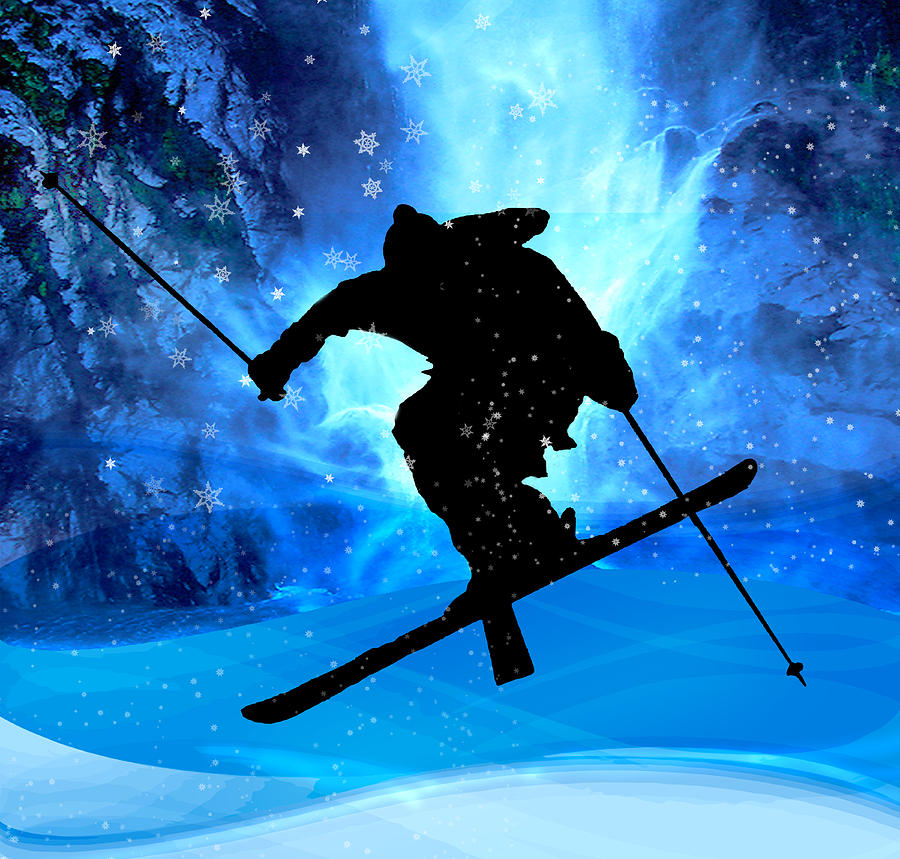This digital artwork features a striking silhouette of a skier mid-jump, with their crossed skis forming an X shape. The skier, appearing as a black shadowy figure, is depicted twisting their body in an expressive manner while gripping ski poles—one pointing up and the other pointing down. The skier is also adorned in a jacket and a beanie. The background is an intense and vibrant blue, interspersed with swirling waves of light and numerous falling snowflakes, giving the scene a dynamic and energetic feel. Flanking the skier are rocky formations, and the entire image is overlaid with white dots and stars of various sizes to mimic falling snow. The bright blue light radiating from behind the skier adds an ethereal touch to this graphic portrayal of a winter adventure.